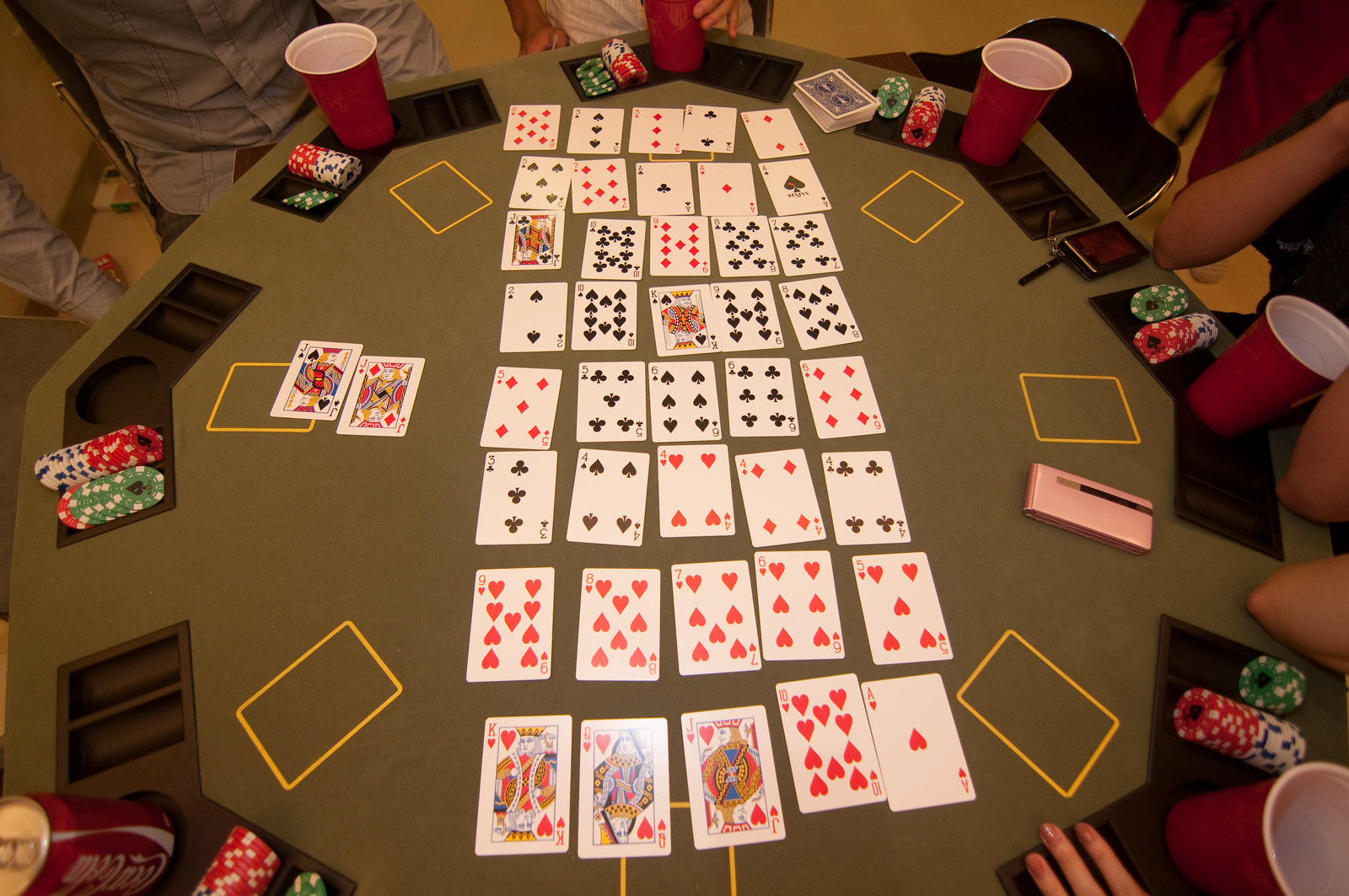This image captures an overhead view of a bustling poker table, accommodating at least six players. The table is neatly organized for a game, with eight rows of five cards each spread out in the center, indicating a detailed and strategic play. Five players are partially visible, signified by glimpses of their attire and body parts. On the left side of the image, an additional place setting is hinted at by the presence of a Coca-Cola can. 

Surrounding the table are various red Solo cups, suggesting that each player has a drink within reach. The table is also adorned with an assortment of poker chips in red, white, black, and green. Intriguingly, a phone with a distinctive pink case lies face-down on the table, hinting at a momentary intermission from digital distractions.

The players are dressed in a variety of outfits, contributing to the lively atmosphere: one man sports a button-up shirt, another prefers short sleeves, and a noticeable presence of red attire adds a pop of color to the scene. Each element in the image collectively encapsulates the camaraderie and intensity of a poker night among friends.